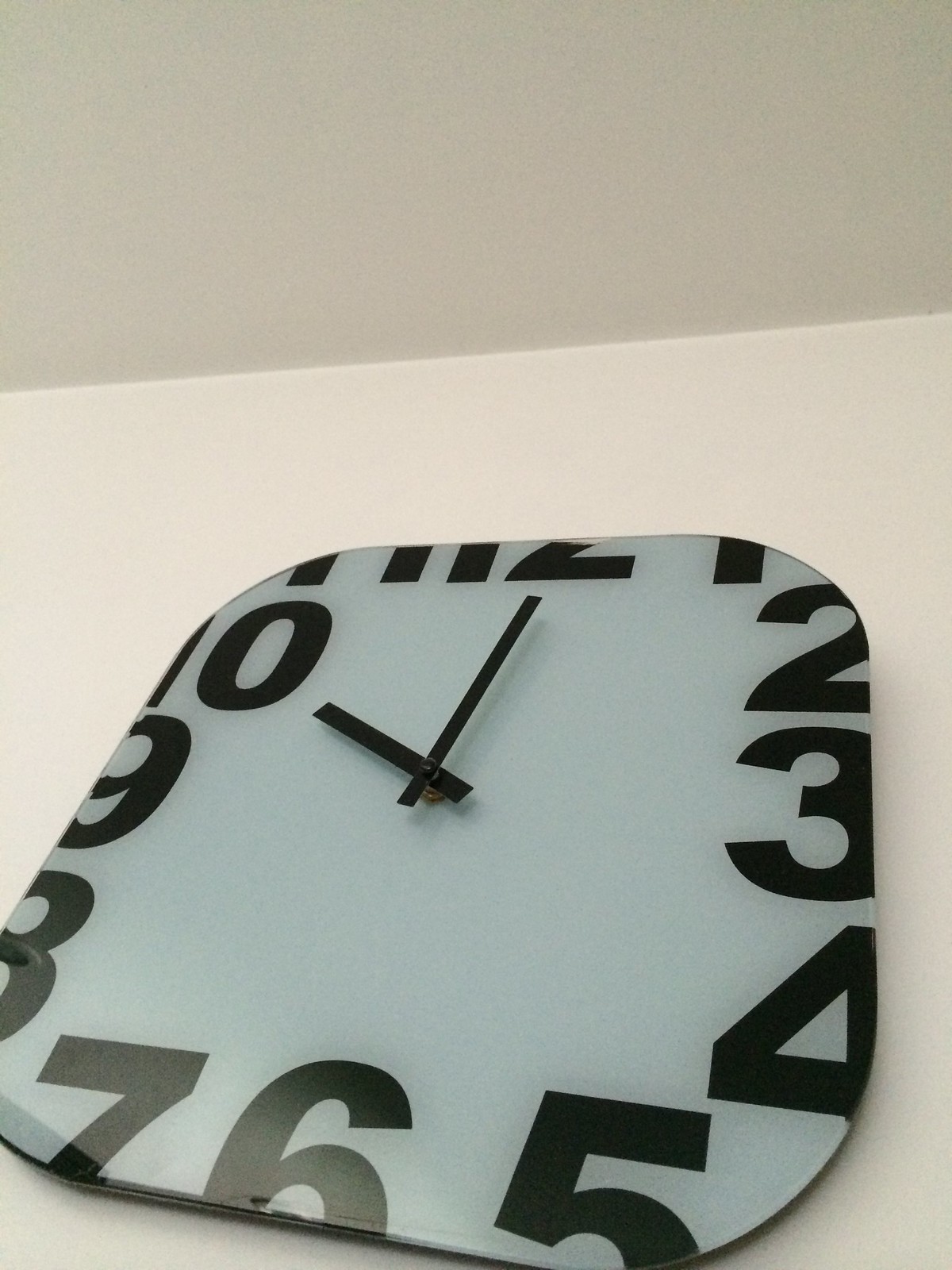This grainy color photograph captures a rectangular clock with rounded edges, mounted on a white wall. The clock, which tilts slightly to the right, features simple, bold, black rectangular hands, positioned to indicate the time is around 12:02 or 10:00, depending on the interpretation of the slant. The hands are secured by a central black screw with a slightly gold rounded base. Its face is an off-white or light grey, contrasted by large, black numbers that are partially cut off at the edges but still entirely legible around the clock's perimeter. This graphic and smooth design of the clock, with numbers appearing printed rather than raised, mounts near the top of the wall where it meets a white ceiling, enhancing the image's clean, minimalist aesthetic.